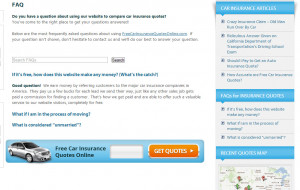A blurry and pixelated image predominantly features shades of white, gray, and blue. In the foreground, there is a partially visible silver car. The lower portion of the image contains a profile with text promoting "Free Car Insurance Quotes Online." An orange rectangle with the text "Get Quotes" is prominently displayed at the center of this promotional banner. The overall quality of the image makes it difficult to discern finer details due to its out-of-focus and pixelated nature.